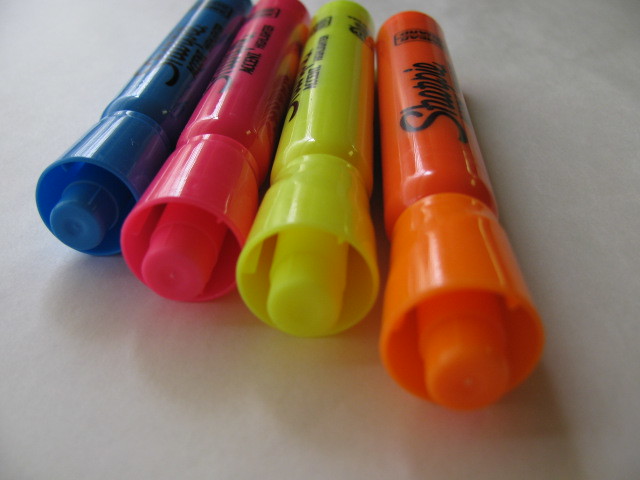In this detailed photo, four Sharpie highlighters are laid out side by side on a white surface. The markers are positioned with their caps pointed towards the camera, offering an almost eye-level view of them. Starting from the left, the colors are blue, pink, yellow, and orange, with the orange highlighter being centrally placed and most prominent. Each highlighter bears the Sharpie logo in black script, clearly visible on their shiny bodies. The caps and bodies match the ink color inside, with the highlighters appearing relatively thick. The lids have a small protruding section designed for stacking the markers on top of each other. The lighting from above creates subtle reflections on the markers, enhancing their glossy appearance, and casts shadows on the white surface beneath them.